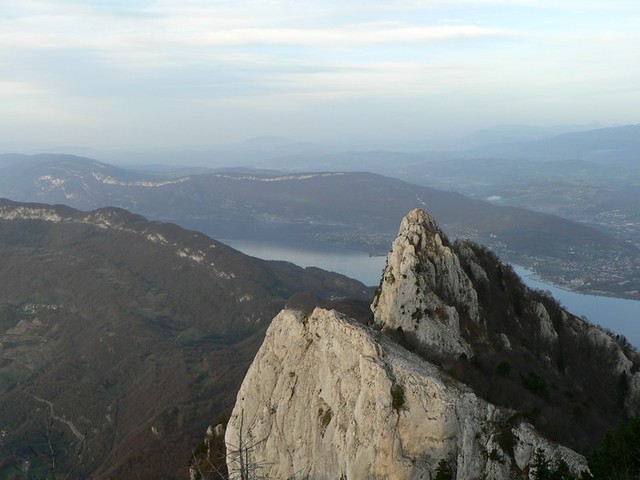This aerial photograph captures an expansive mountainous region characterized by a series of distinct rock formations and a flowing body of water. Dominating the foreground are two prominent, gray rocky peaks, situated toward the bottom of the image. These peaks face leftward, with their highest points reaching the upper right center and sloping downward to the lower right corner.

To the left of these peaks, a tree-covered mountain with more rounded, darker summits stretches into the scene. Nestled between the mountain ranges lies a serene, blue river or large lake, which meanders from the center left to the right edge of the photograph.

In the backdrop, another tree-clad mountain range ascends gently, appearing misty and distant. Faintly visible behind this is an even farther mountain range, shrouded in fog and adding layers to the depth of the landscape.

The upper portion of the image is dominated by a partly cloudy sky, featuring a mix of white and gray clouds that blanket the blue expanse. The colors in the photograph vividly depict the natural elements: the lush green of the trees, the tranquil blue of the water and sky, the light and dark tones of the rock formations, and the brown patches of land interspersed throughout the scene. This picturesque setting encapsulates the raw and serene beauty of a remote mountainous area.